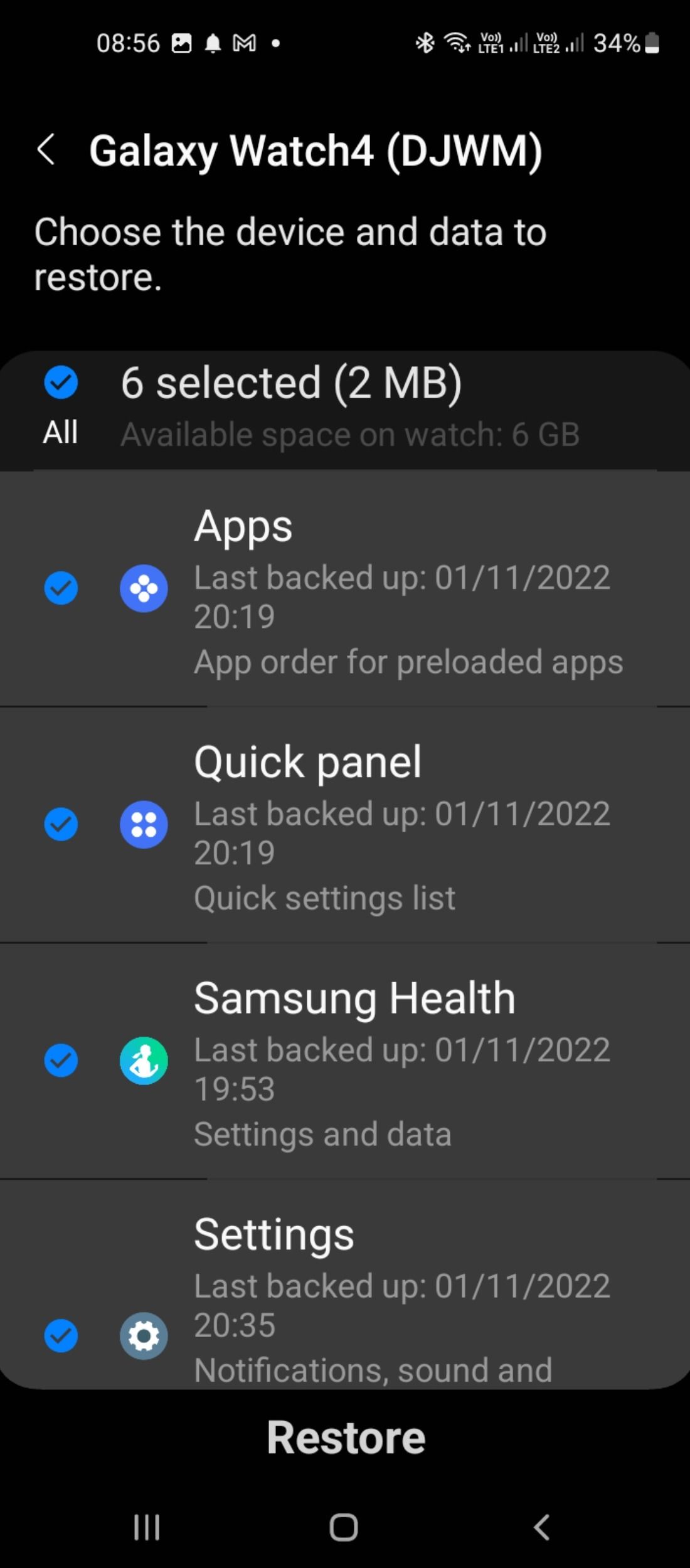A detailed screen capture of a mobile application in night mode is shown on a smartphone. The background is rendered in shades of gray and black, with white text providing clear contrast. At the top of the screen, the status bar displays various statistics and control panels, including the time, which reads 8:56, and the battery level at 34%. Below this, the text "Galaxy Watch 4 (DJWM)" is prominently featured in white.

Underneath this header, the screen instructs, "Choose the device and data to restore." A gray window with rounded corners displays the message "6 selected, 2 MB." The panel lists four selected items, each indicated by a blue checkmark on the left and a corresponding small round icon. The top two icons are blue, the third is green, and the lowest is gray. These items represent "Apps," "Quick Panel," "Samsung Health," and "Settings."

Each item’s header text is in white, while the details beneath, including the last backup date, are displayed in gray. At the bottom of the screen, the word "Restore" appears in white text. Below this are three navigation buttons: the left one with three vertical lines, the central button resembling a square with rounded edges, and the rightmost one displaying a left-pointing arrow.